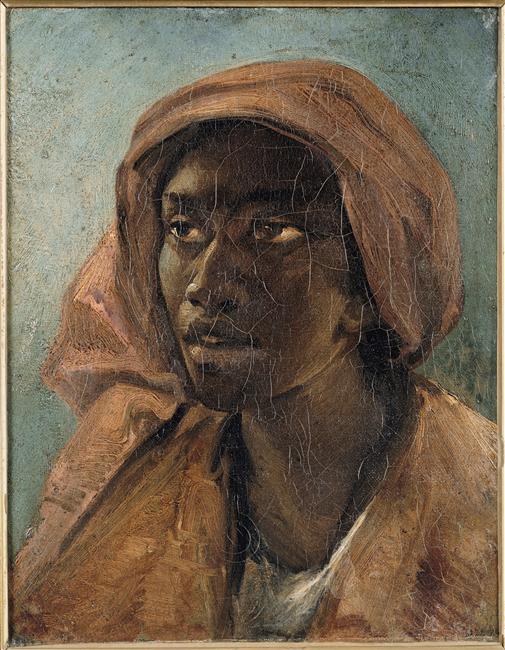This detailed painting portrays a young African American woman seated against a muted blue-gray and greenish background. Her large, expressive brown eyes are looking to the left, accompanied by a slightly open mouth revealing her top teeth, contributing to an ambiguous, perhaps sad expression. She wears a headscarf of an orangey-brown hue that wraps around her head and gathers at her neck on the left side, matching the cloak or dress she is wearing. Beneath this, a light-colored blouse, visible at the neckline, forms a V-shape. The painting's surface showcases intricate crackling, adding to its textured, aged appearance. Framed by a thin, elegant gold border, this artwork captures a gentle, contemplative moment.